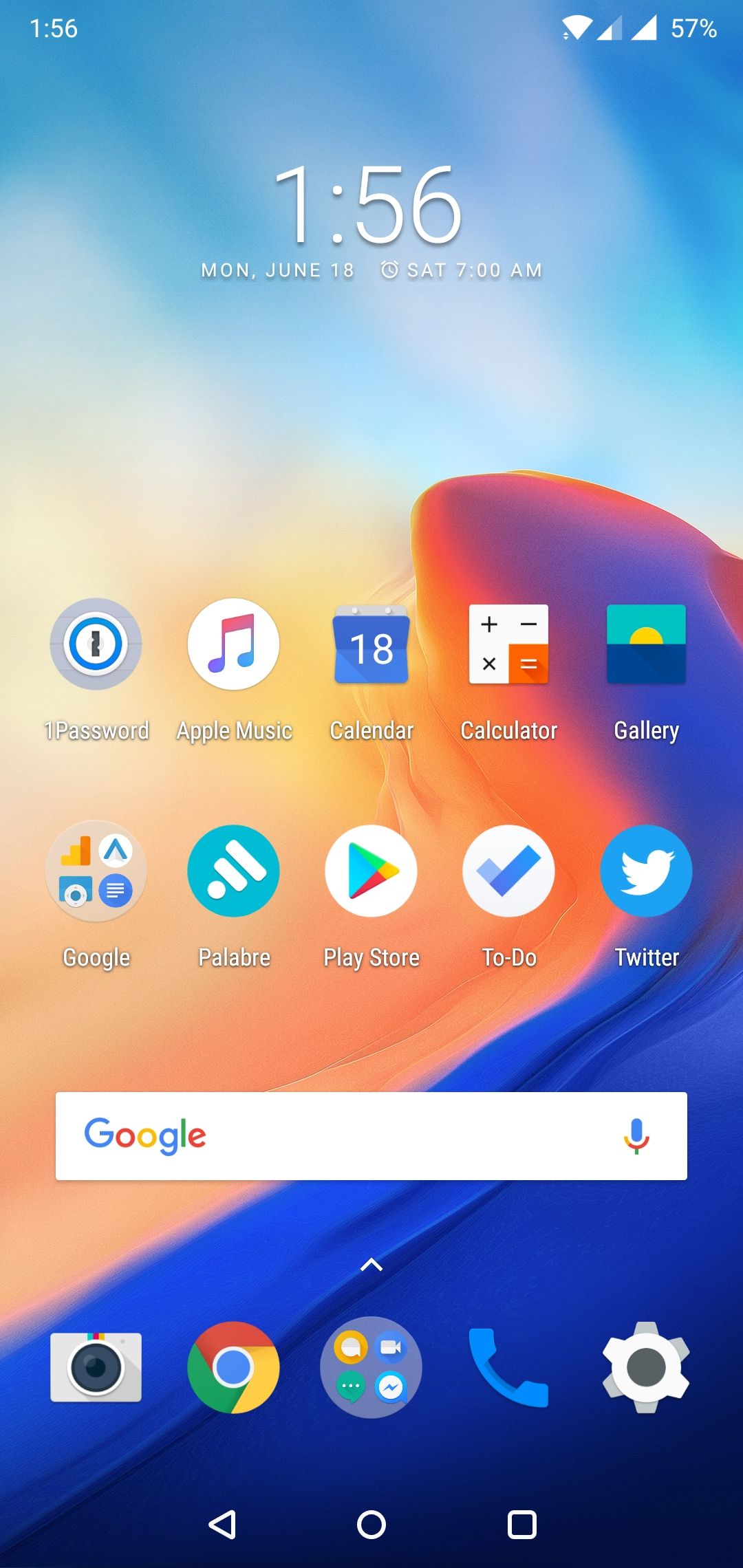This image showcases a smartphone with a visually captivating background featuring a swirling motif. The upper section of the background depicts a sky-effect intertwined with a sandstorm, blending vibrant hues of yellows, oranges, and purples, cascading down to an indigo-dominated corner. The date and time displayed on the phone reveal that it is Monday, June 18th, with an alarm set for Saturday at 7 a.m.

The phone's home screen displays a variety of app icons neatly arranged. It includes:

1. **Password** - An app icon unfamiliar to the narrator.
2. **Apple Music** - A popular app for music enthusiasts.
3. **Calendar** - Showing the date as June 18th.
4. **Calculator** - With standard mathematical function icons.
5. **Gallery** - This icon seemingly resembles a flag with a turquoise field and a yellow circle, partly obscured by a gray overlay.
6. **Google** - The well-known search engine's app.
7. **Palabra** - Presumably a language or word-related app.
8. **Google Play Store** - For downloading apps.
9. **To-Do List** - For task management.
10. **Twitter** - The social media platform icon.
11. **Camera** - For photo and video capture.
12. **Google Chrome** - The web browser.
13. **Media App** - Possibly referring to an app for multimedia.
14. **Phone** - For making calls.
15. **Settings** - The gear icon for configuring the device.
16. **Search Screen** - Google search bar set up for easy access.

The image combines aesthetic appeal with practical elements of a phone's interface, suggesting a balance between functionality and visual delight.